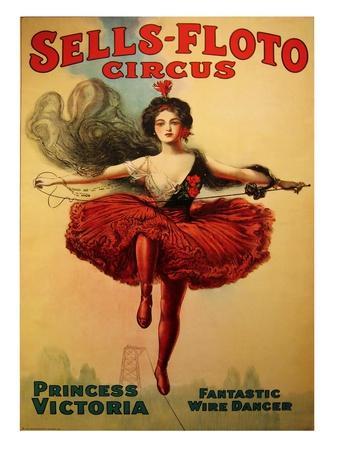This vintage illustrated advertisement for the Sells Floto Circus prominently features Princess Victoria, described as a "Fantastic Wire Dancer." At the very top, large red letters spell out "Sells-Floto Circus." The bottom left corner names the star performer, Princess Victoria, while the bottom right highlights her skill as a "Fantastic Wire Dancer."

In the center of the poster, Princess Victoria is depicted performing a dazzling tightrope act. She strikes a dramatic pose, standing on one leg on the wire. She wields another wire in her hands, perhaps to be swung around in her performance. Her attire is striking: a flowing red dress that cascades from a V-neck top over her chest into a large red frilly skirt, complemented by red tights. She also has wispy, black hair adorned with a small red accessory, flowing to the left like smoke. The background suggests an old-timey, rustic scene with a weathered yellow hue, reminiscent of posters from the 1930s or 1940s, lending it an antique charm. The overall design, with its historical and vivid details, emphasizes the thrilling spectacle that Princess Victoria promises to deliver.